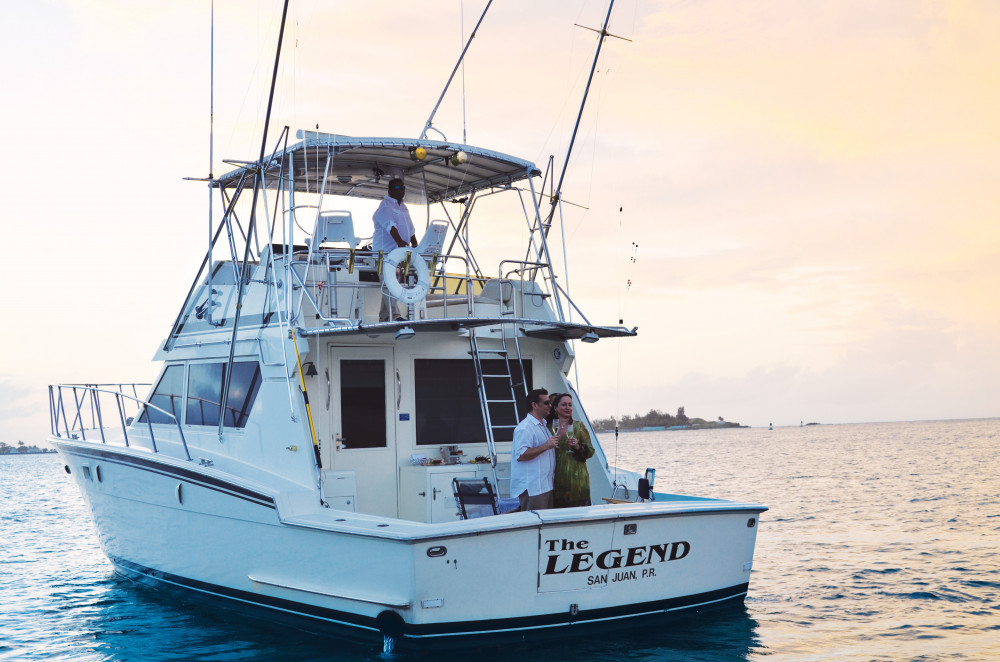The photograph, taken during daylight with the golden hues of an approaching sunset, captures a large, two-story yacht named "The Legend" from San Juan, Puerto Rico, prominently positioned in the scene. The sky occupies almost two-thirds of the image and is slightly cloudy with a tint of orange, reflecting the sunset. The yacht is primarily white with sleek black or blue trim lines along its border and lower-edge, and it bears the name "The Legend" in large black text centered on the front, with "San Juan, PR" in smaller letters below.

On the top deck, a man in a white long-sleeved shirt with sleeves rolled up, short black hair, and mirrored sunglasses stands beside a life preserver, looking out over the ocean. The top deck also features several metal projections and a protective roof over the seated area. On the lower deck, nearer the front of the yacht, a couple – a man and a woman – is seen standing close together, both holding champagne glasses. The man, dressed in a white short-sleeved shirt and khaki trousers, has his arm around the waist of the woman, who is wearing a long-sleeved green dress and has dark brown hair.

The background reveals calm blue waters and a distant island with trees and small buildings near the shore, enhancing the serene atmosphere of the scene. The boat's well-defined structure includes tinted windows and a door leading into the main cabin, suggesting an enclosed space for shelter against the elements. The overall composition of the image emphasizes the luxurious and leisurely setting on a yacht, with each person on board enjoying the picturesque ocean view.